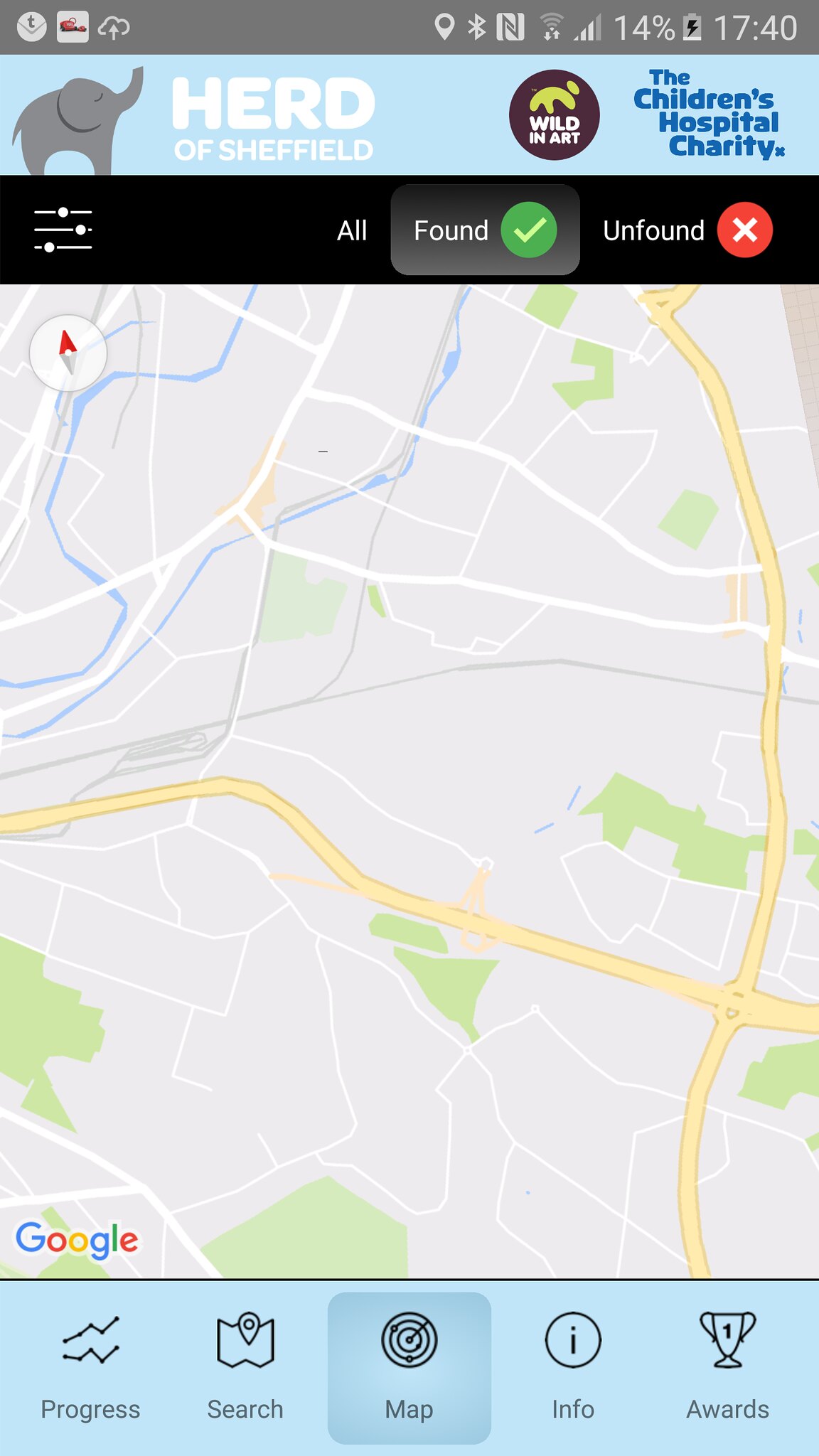A smartphone screen displays a Waze navigation app prominently. At the top section, typical smartphone interface elements are visible, including icons and the time displayed as 7:40. Directly beneath this is a rectangular advertisement featuring a blue profile of an elephant with the text "Herd of Sheffield" and "The Children's Hospital Charity" to its right.

The central area of the screen showcases the Waze map, which is predominantly gray. A major highway runs from the lower right edge, extending vertically to the upper left edge. In the upper portion of the screen, another section of highway enters from the center-left edge, takes a slight upward right turn, then a downward right turn, and finally intersects with the primary highway.

Additional roads, depicted as diagonal and horizontal lines, are mostly situated in the upper half of the map. In the upper left corner, a simple compass icon is located with the north point slightly to the left.

At the bottom of the screen, a light blue ribbon features various icons. Below these icons, there are five options: "Progress," "Search," a highlighted "Map" in the center, "Info," and "Awards" on the far right.